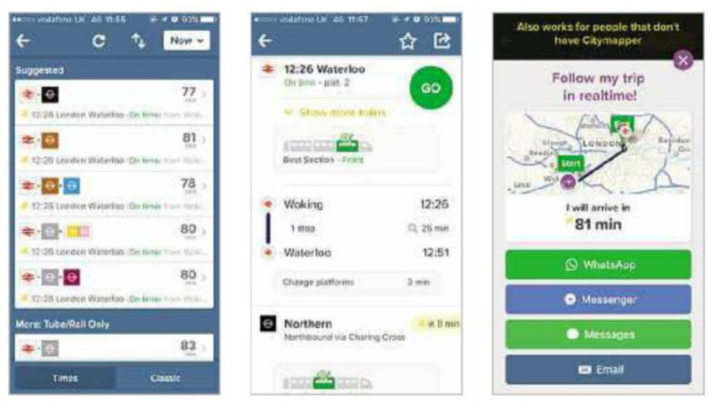### Detailed Descriptive Caption:

The image comprises three sequential screenshots from a mobile application. 

**First Screenshot:**
- The battery icon indicates a 93% charge.
- The top bar includes a left arrow, a refresh symbol, an up-and-down arrow, and a "New" label.
- Five lines of information are displayed under a section titled "Suggested".
- There is a heading or content labeled "More to/ Rail only. Arelli" (which appears as "R-E-L-L").
- The bottom section features the text "1 MES" and an option labeled "Classic or Times". "Classic" is displayed on a dark blue rectangle, while "Times" is highlighted on a light blue rectangle.

**Second Screenshot:**
- The battery charge remains at 93%.
- The top bar includes a left arrow, a star icon, and a share button.
- The screen shows a time or location label "1226 Waterloo" together with a restaurant name, "The Greens to Go".

**Third Screenshot:**
- The main focus is on a text reading "Follow my trip in real time" highlighted in purple. 

Together, these screenshots illustrate user navigation through different sections of an app, likely involving transportation or location-based services.